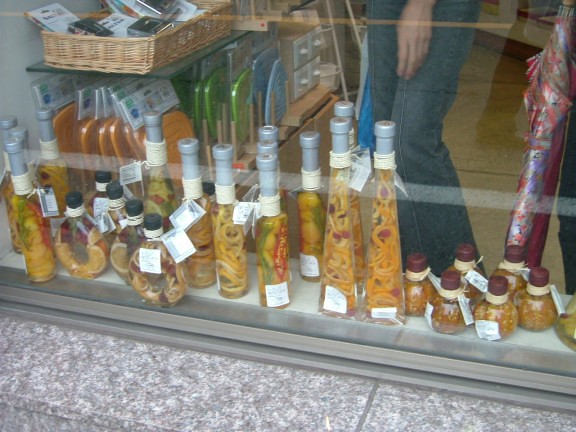This photograph captures an exterior view of a store window, focusing on a display of various infused olive oils and vinegars. The bottom of the image showcases a concrete ledge just outside the store, transitioning into the metal bottom edge of the window frame. Within the window, arranged on a shelf, are numerous glass containers and bottles filled with a variety of infused oils. The bottles differ in shapes and sizes, from tall, clear bottles with silver tops containing stringy foods, to squat, oval-shaped containers with black and red tops. These vessels hold a colorful array of ingredients such as peppers, lemons, chilies, onions, spices, and olives, each contributing to the rich, visual tapestry of the display. In the background, the legs and hand of a person clad in jeans are visible, adding a subtle human element to the scene. Toward the right of the bottles, there is a bolt of red and silver fabric, while on the left, shelves mounted against the wall hold a basket and other lined-up items, further enriching the detailed composition.